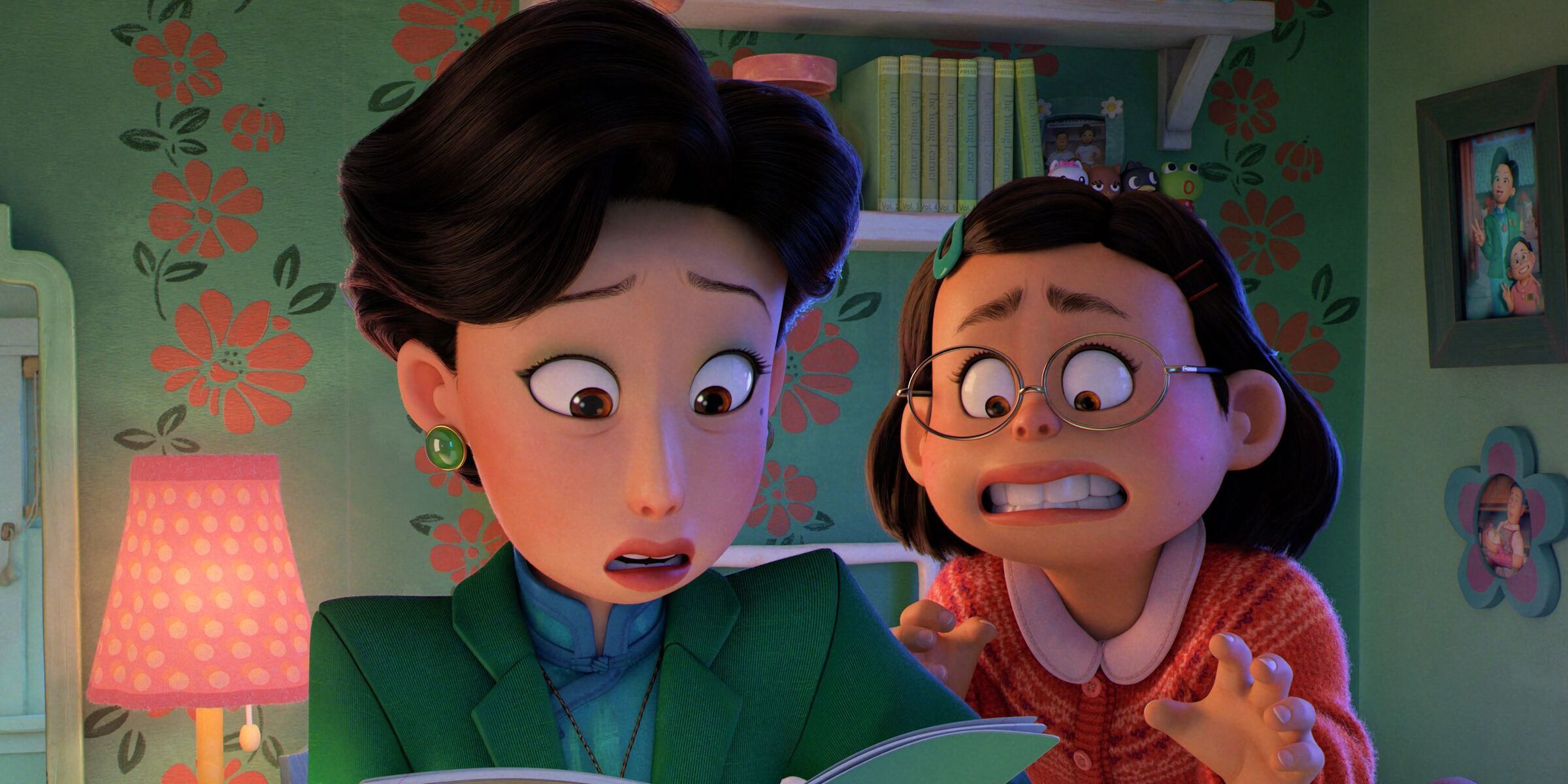This image is a detailed still from the animated 3D movie "Turning Red." The scene features two characters, a woman and a young girl, who seem to be in a living room with Chinese aesthetic influences characterized by soft blue, pink, and green tones. The woman, situated on the left, has short brown hair, a formal green suit, and matching earrings. She appears to be in shock as she looks down at a green book that is mostly off-camera. The girl on the right, who has a younger and nerdier appearance with glasses, a red sweater, and a somewhat chubby build, seems concerned or hesitant about the situation. Both characters are drawn with expressive faces that clearly convey their emotions. In the background, there is floral wallpaper, a lamp with light pink polka dots, a bookshelf, and several pictures on the wall, contributing to the homely and culturally rich setting of the scene.